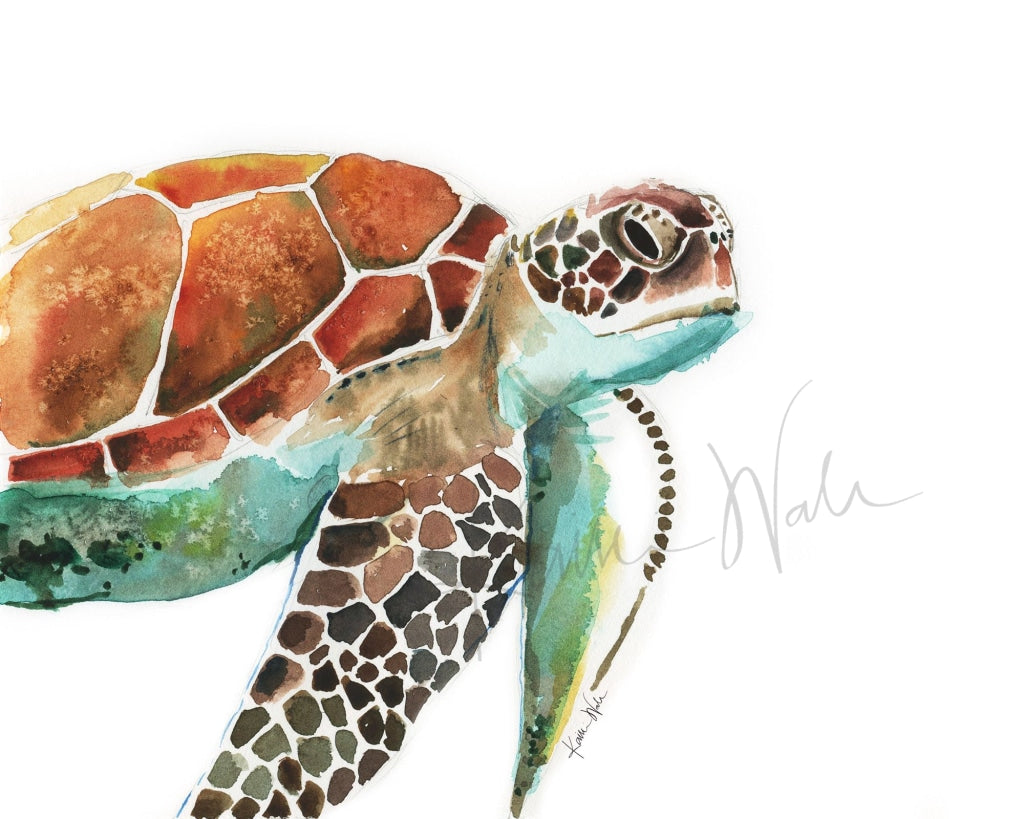This is a detailed watercolor illustration of a multicolored sea turtle set against a white background. The turtle is depicted with a rich mixture of colors, primarily browns, yellows, greens, blues, and teals. The shell is adorned with warm hues such as red, orange, and light brown, featuring a pattern that resembles a series of scaled or rock-like designs. The head and front flippers are dark brown with noticeable scales, and the black eyes add a touch of realism to the face. The underside of the turtle is shaded in cooler tones, including teal, blue, and green. There are two signatures from the artist; one larger and in cursive near the turtle's flipper, and a smaller one positioned at the bottom of the image. Additionally, a watermark is visible at the bottom of the illustration, emphasizing the artistic value of the piece.